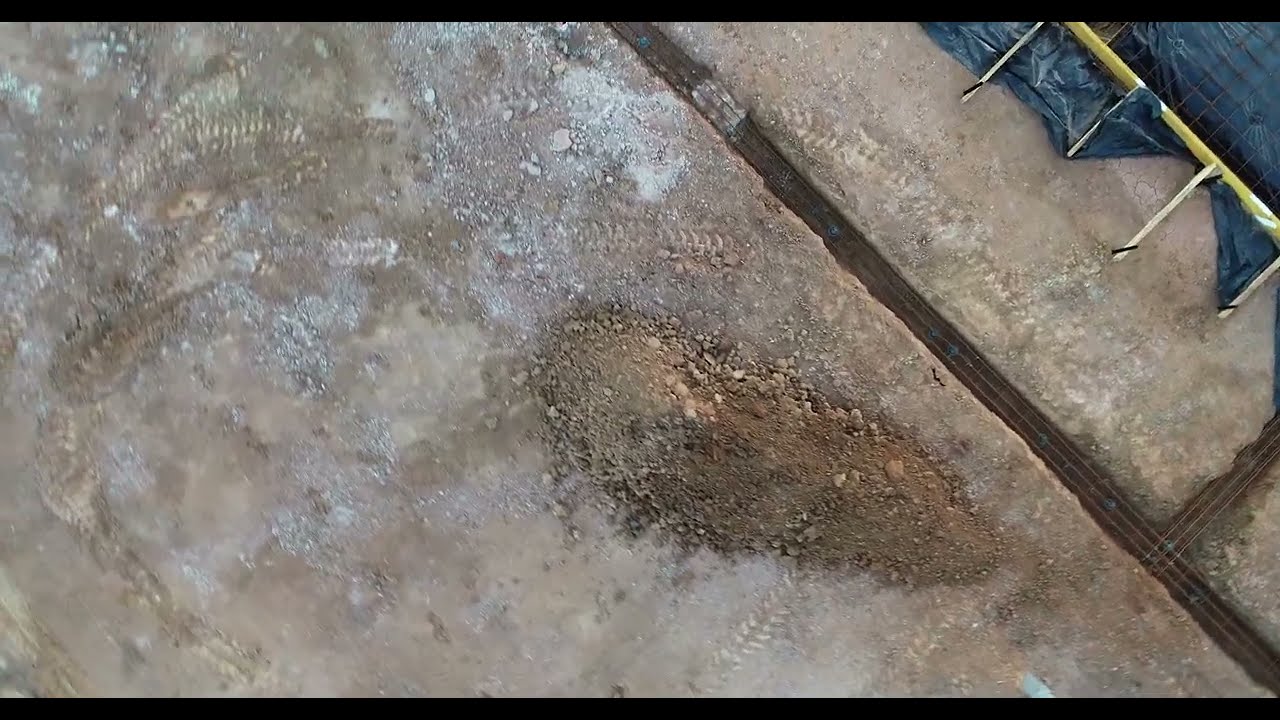This image appears to be taken from above, capturing a disorganized construction or loading site. The photograph is slightly diagonal, adding a sense of disorientation. The focal point is a freshly dumped pile of dirt, centrally located but slightly to the right and bottom of the image. This mound of earth is light brown on top, transitioning to darker brown towards the right. The surrounding ground is dirty, primarily brown with splotches of white, crisscrossed by tire treads and possibly footprints indicative of construction vehicles.

In the upper right corner, there is a noteworthy structure consisting of a metal grate or grid supported by yellow-brown barriers. Behind this barrier is a blue tarp or plastic sheeting, possibly used to cover or protect materials. Below this structure, a narrow trench runs diagonally from the top center to the bottom right of the image, intersecting with a T-junction. Thin wires or metal rods, possibly three in total, are visible at the bottom of the trench. 

To the right of the dirt mound, there is what appears to be a road or pathway, darker brown in color and marked by tracks from heavy equipment. The image also features sections of brick dividers, further segmenting the area. The overall scene is cluttered, with elements indicative of an active, yet untidy, construction or material handling site.